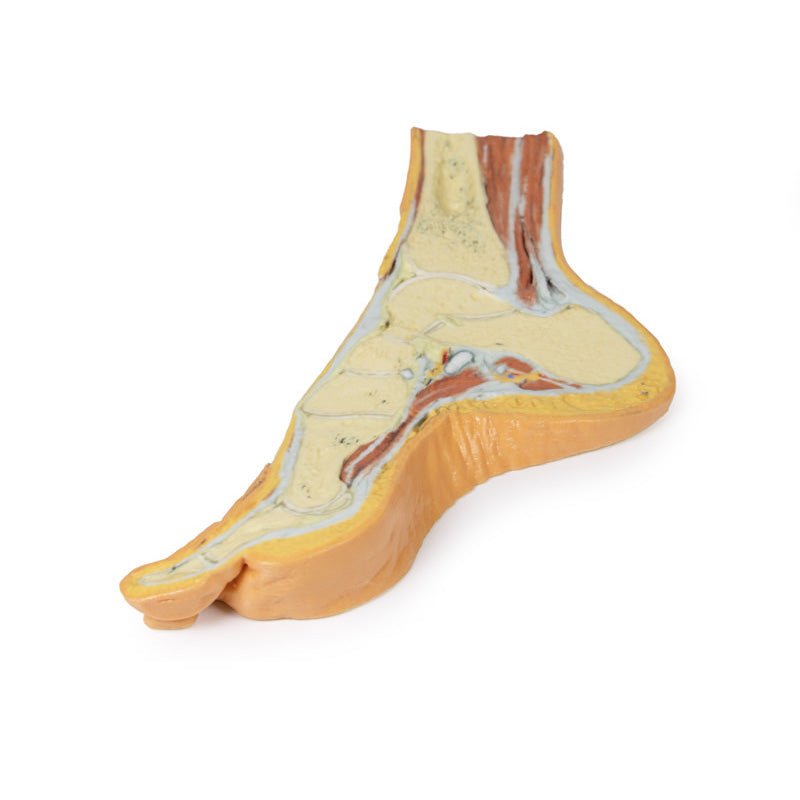This image is a detailed, color photograph of a cross-section model of a human foot. The model is sliced in half along its length, with the big toe prominently pointing to the left. The exterior skin of the foot is depicted in a peach or tan color, while inside, various anatomical structures are visibly detailed. The high arch of the foot is notable, and the cross-section extends slightly past the ankle.

The internal structures showcase the muscles, tendons, bones, and cartilage with distinct colors for each: the muscles are a reddish pink to dark red, stringy in texture; the bones are cream or yellowish in hue; tendons and ligaments appear in light blue; and the cartilage is white. There is also a layer of dark orange-yellow fat just beneath the skin.

Two white circles are visible within the cross-section, possibly representing anatomical points of interest. The model appears to be made of plastic and is likely intended as an educational tool, probably for an anatomy class, to illustrate the complex internal structures of the foot.